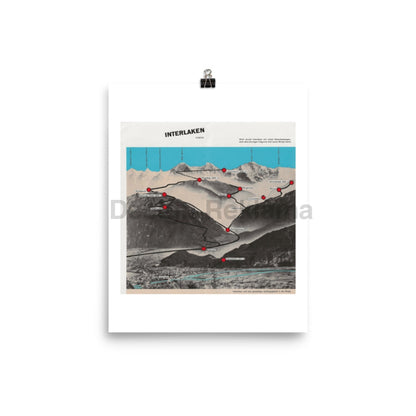This image depicts a low-resolution stock art illustration of a ski resort map labeled "Interlaken," a well-known resort town in Switzerland. The primary focus is a white mountain with numerous red dots and zig-zagging lines that likely indicate various ski routes, possibly highlighting different paths for skiers of varying skill levels. The top of the image prominently features the name "Interlaken" in bold black letters. The background shows a vibrant, artificial blue sky, giving the scene a more distinct appearance. Additionally, a small amount of illegible text, possibly the watermark of a stock image website not in English, is present on the image. The entire illustration appears to be a piece of paper held up by a typical office paper clip, with a blue body of water, possibly a lake or river, running adjacent to the mountain at the bottom edge of the picture.